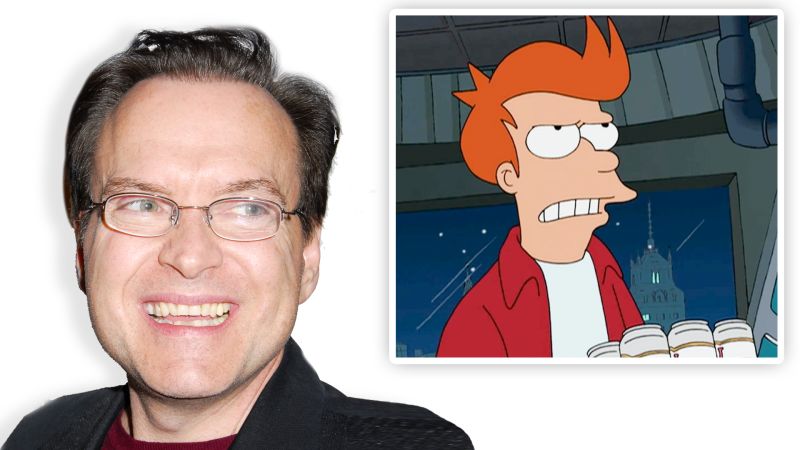This image features two distinct pictures side-by-side on a solid white background. On the left is a close-up photograph of a middle-aged Caucasian man with blue-gray eyes and dark, possibly brown, hair. He is smiling warmly with his teeth showing, and is wearing glasses, a red shirt, and a dark gray or black jacket. His image has been photoshopped against a plain white backdrop. To the right of this man's photo is an image from the animated series Futurama, depicting the character Fry. Fry, with his trademark orange hair, is wearing a red jacket over a white shirt and is holding a six-pack of canned beverages, presumably beer. He is scowling and looking to the right, with a detailed background showing a night sky, cityscape, and part of a window frame visible through which the city can be seen. The juxtaposition of these images suggests a possible connection between the man and the animated character, potentially implying that the man could be the voice actor for Fry.